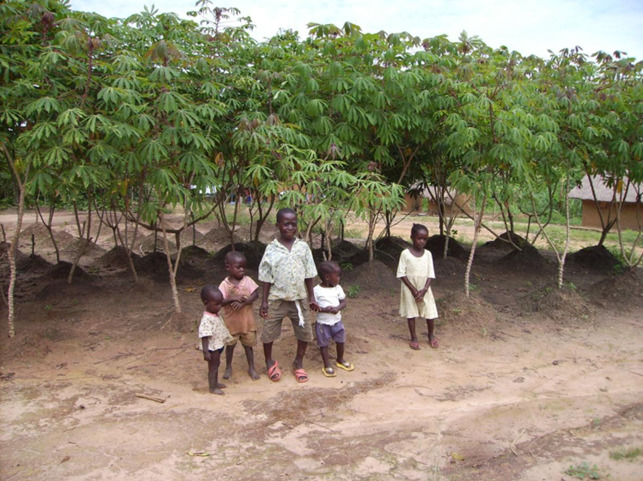The photograph captures a group of five African children standing outdoors under a slightly cloudy blue sky. The scene is set on a dirt road, with some sparse grass visible in the foreground, flanked by recently planted, thin-trunked trees with green leaves. The children, who appear to be very young, dressed for warm weather with short sleeves, shorts, or a dress, and are likely in preschool or early elementary grades. 

The first child wears a beige shirt with blue shorts and is barefoot. The second child, also without shoes, has an orange shirt and shorts that show signs of dirt, indicating playful activity. The tallest child stands out with a white button-down shirt, khaki pants, a visible drawstring, and pink flip-flops. Another child, possibly a girl, with braided hair, sports a white shirt, blue shorts, and yellow flip-flops. Finally, a girl in a yellow dress holds something in her hands, with pink flip-flops on her feet.

All the children, with dark brown skin, suggesting their African heritage, seem to be posing for the camera but are not looking directly at the photographer. In the background, beyond the trees, there are glimpses of traditional huts, adding to the rural ambiance of the scene.